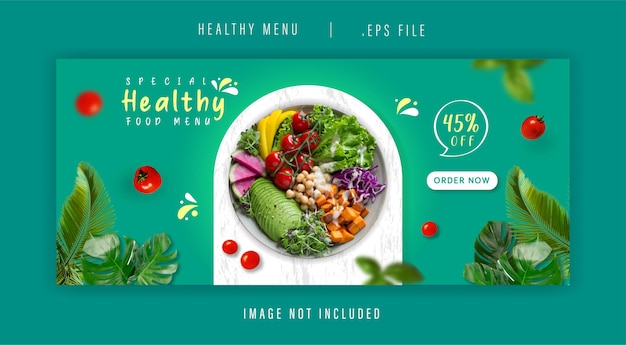This promotional image features a blue background adorned with a design of tomatoes and various plants. At the center, there's a photograph of a plate filled with a vibrant salad, showcasing an array of fresh vegetables, including a visible lemon and other green vegetables. The text highlights a "Special Healthy Food Menu" with an attractive offer of 45% off. The call-to-action, "Order Now," is prominently displayed in a turquoise blue color on a white rectangular button. Note that the image in the promotional text states "image not included." The file is available in EPS format.